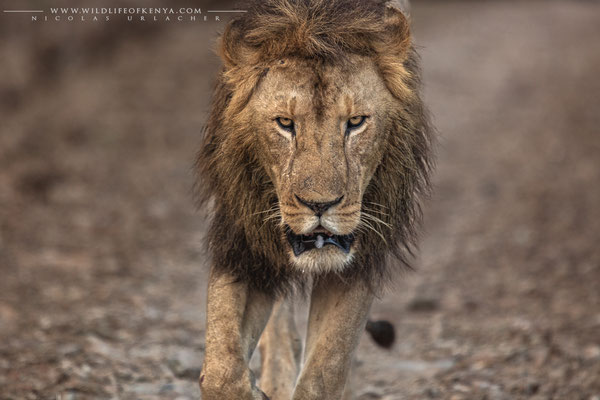This striking close-up photo captures a male lion with a textured, scraggly mane and light brown fur, almost a golden bronze, trotting directly towards the camera. His piercing eyes are fixed on the viewer, with his mouth slightly open and one paw lifted mid-stride. The soft lighting and possible use of a soft focus filter lend a gentle touch to the image. In the blurred background, creating a bokeh effect, the indistinct grayish-brown strata of rocks or dirt add contrast, ensuring the lion remains the photograph's undeniable focal point. At the top left-hand corner, the web address www.wildlifeofkenya.com is displayed, followed by the name Nicholas Urlacher, presumably the photographer. The lion, centered vertically in the shot, appears almost to be filling the entire frame, suggesting the probable use of a telephoto lens to capture this majestic creature up close while maintaining a safe distance.